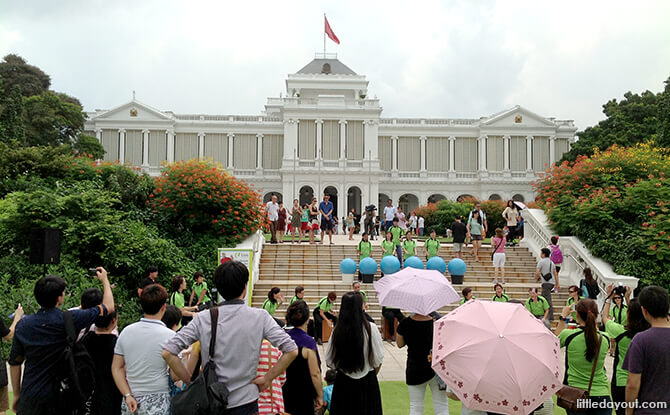The image depicts an outdoor event at what appears to be a large, white marble building with columns and arched windows, resembling a capitol building. A red flag is perched atop the domed, ornamented roof. In the foreground, several photographers are capturing the scene, two of them holding pink umbrellas to shield from the sun. One man, with a bag slung over his left shoulder, is notably positioned on the far left, taking a picture. 

In the middle ground, a group of people wearing identical green and black striped shirts are prominently featured. At least four of these individuals are engaged in a performance, appearing to pound on drums with blue balls situated in front of them, scattered on the steps. Behind them, additional participants and onlookers are visible, some wearing similar uniforms, while others are dressed more casually in shorts and short sleeves, indicating pleasant weather. The steps leading up to the building are flanked by green and orange foliage, adding a colorful backdrop to the scene.

The lower right corner of the image contains the website littledayout.com in white print, suggesting this photograph was taken during a lively community event or festival. With people positioned at various levels of the steps and the lawn, the image captures the energetic atmosphere of the event, framed by lush trees on both sides.